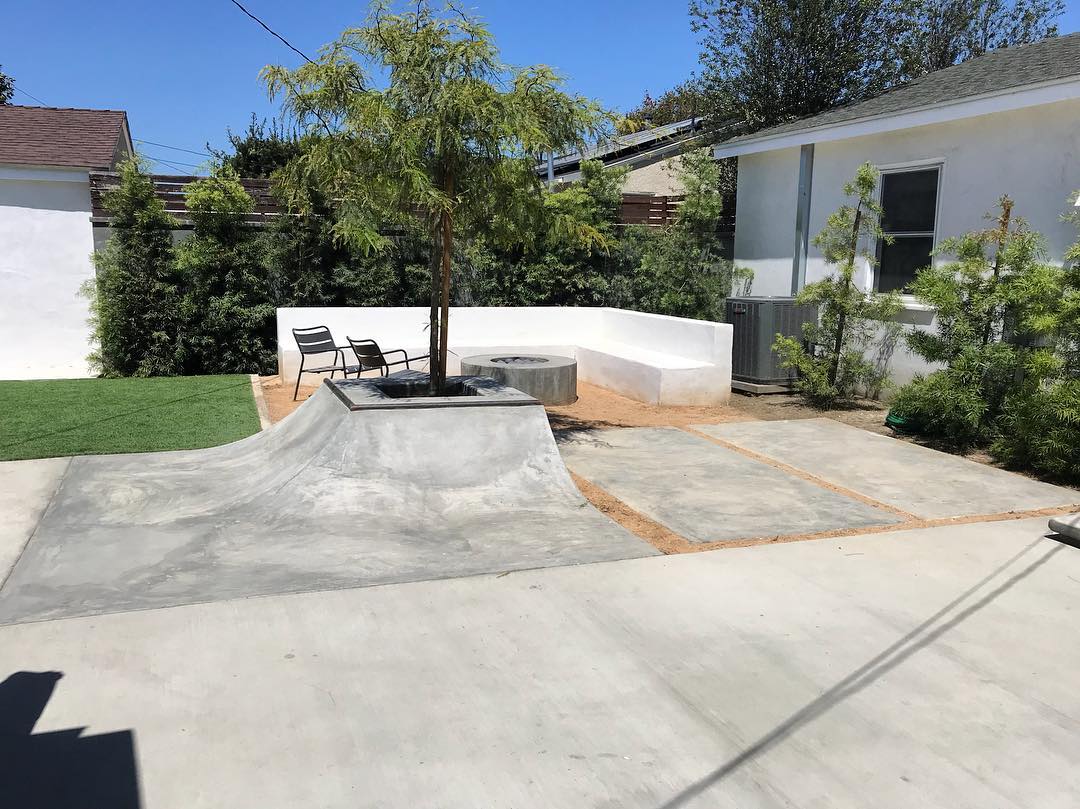The image depicts a backyard patio primarily covered in concrete. Central to the scene is a raised concrete planter that houses a prominent tree, which also functions as the top of a skateboard ramp. This planter is bordered by some breaks in the concrete, revealing the dirt beneath. The area also features a seating arrangement with two chairs and an L-shaped white concrete bench positioned around a fire pit, all set on a dirt or sandy section separate from the main concrete pad.

Bordering the patio are two buildings. The house on the right has an air conditioning unit affixed to its exterior and features a window with three additional plants lined up beside it. To the left, another house or shed connects to the first building via a fence, along which more small trees are planted. Adjacent to this fence, there is further seating with concrete poured seating and a concrete fireplace, enhancing the patio's multifunctional outdoor living space.